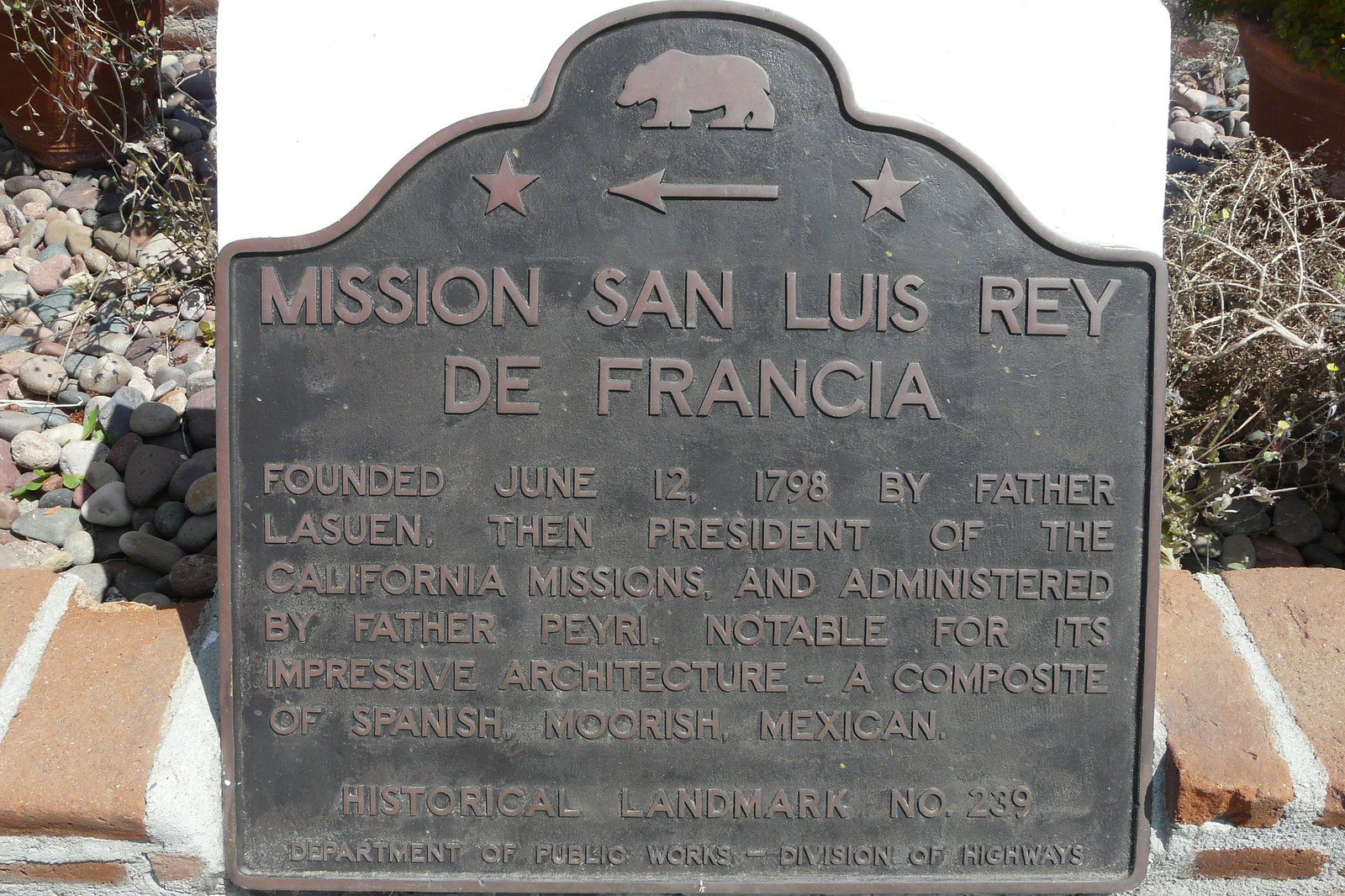This image is a color, landscape-oriented photograph capturing a historical plaque dedicated to Mission San Luis Rey de Francia, a notable mission in the state of California. The plaque is made of wrought iron with a dark background and light bronze lettering. At the top of the plaque, there is a California Grizzly bear facing sideways, an arrow pointing left, and a star on each side of the arrow. Below the bear, the text reads: "Mission San Luis Rey de Francia," followed by, "Founded June 12, 1798 by Father Lasuen, then president of the California missions and administered by Father Perry." The plaque highlights the mission's impressive architecture, a blend of Spanish, Moorish, and Mexican styles. It is designated as Historical Landmark Number 239 by the Department of Public Works, Division of Highways. The plaque is mounted on a white stone set within a brick wall, with gravel and planted shrubbery visible behind it. This photograph exemplifies a style of photographic representational realism.